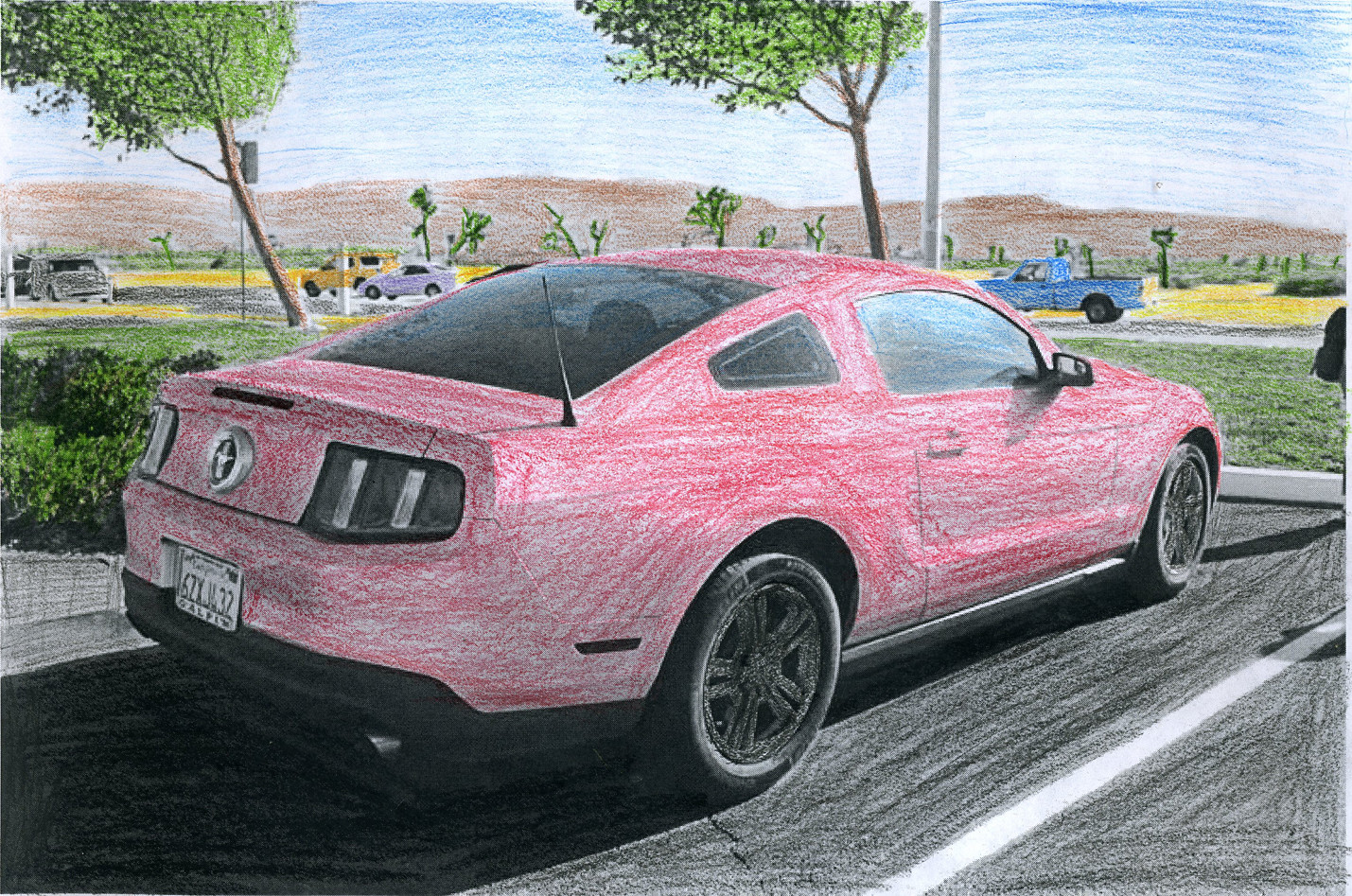This crayon drawing depicts a vivid and playful scene centered around a pink Mustang, positioned prominently in the foreground. The Mustang, a two-door model, features the iconic Mustang emblem on the back, along with a license plate that resembles a California plate, reading something akin to "CZ X??? 32". Despite the car originally being white, it has been enthusiastically colored red with crayons, including detailed accents like black wheels and tires, though notably missing hubcaps.

The car rests on a black asphalt surface, highlighted with black crayon, which leads up to a yellow stripe and a gray cement-colored bumper block. In the scene's foreground, green grass and a narrow gray road add contrast and depth. Moving towards the left side of the drawing, a variety of other vehicles are depicted, including a blue pickup truck directly in front of the Mustang, and further left, a silver coupe and a yellow pickup truck with a canopy.

The background features several trees, a tall light pole, and a distant landscape composed of brown hills under a blue sky. Additional details include a scattering of shrubs to the far left of the car, contributing to the detailed and colorful environment that the artist has created.